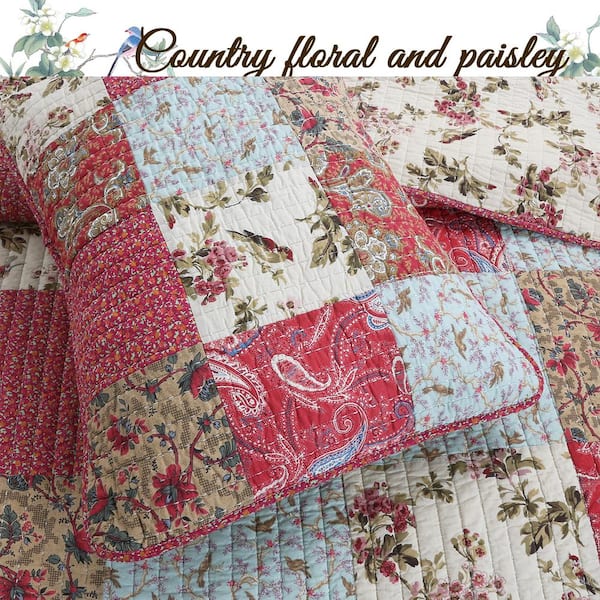The image features an intricately designed quilt accompanied by matching pillows, set against an advertisement or flyer background. Dominating the top section is a white field adorned with white flowers and a blue bird with a pink belly perched on some leaves. This area also contains the words "country, floral, and paisley" written in a cursive brown font. The quilt and pillows showcase an array of patterns primarily in shades of pink, crimson, and white, accented with green. Each section of the quilt boasts a variety of floral prints, red bandana designs, and paisley motifs. Notably, one large block in the center of the quilt features a bird, and several other blocks also include bird illustrations. The quilt exudes a rustic, country charm much like those traditionally handmade, suggesting high-quality construction and attention to detail.